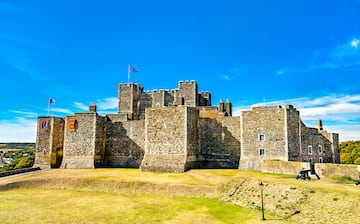The image showcases an old, imposing castle made from gray and brown stone, giving it a distinctly aged appearance. The castle, which is square-shaped, features multiple towers and boxy rectangular structures protruding from its sides. The tallest tower, located at the center, is adorned with a single flag at its peak, while another flag can be seen on a tower on the left side of the building. Both flags add a touch of color against the predominantly stone-gray facade. Nearer to the entrance, additional flags, including one with orange and yellow hues and another that is blue, hang on the castle walls.

In front of the castle, a well-maintained grassy area stretches out, indicative of freshly mowed, lush green grass. This grass-covered terrain is slightly hilly, adding to the picturesque nature of the scene. The vibrant blue sky above, dotted with a few fluffy white clouds, complements the well-lit daytime setting. Sunlight bathes the entire scenery, illuminating the castle's ancient stonework and the surrounding landscape. The photo, although taken from a distance and of low quality, still captures the intricate details, including the potential moss or mold marking the long-standing walls, signifying the castle's historical authenticity.